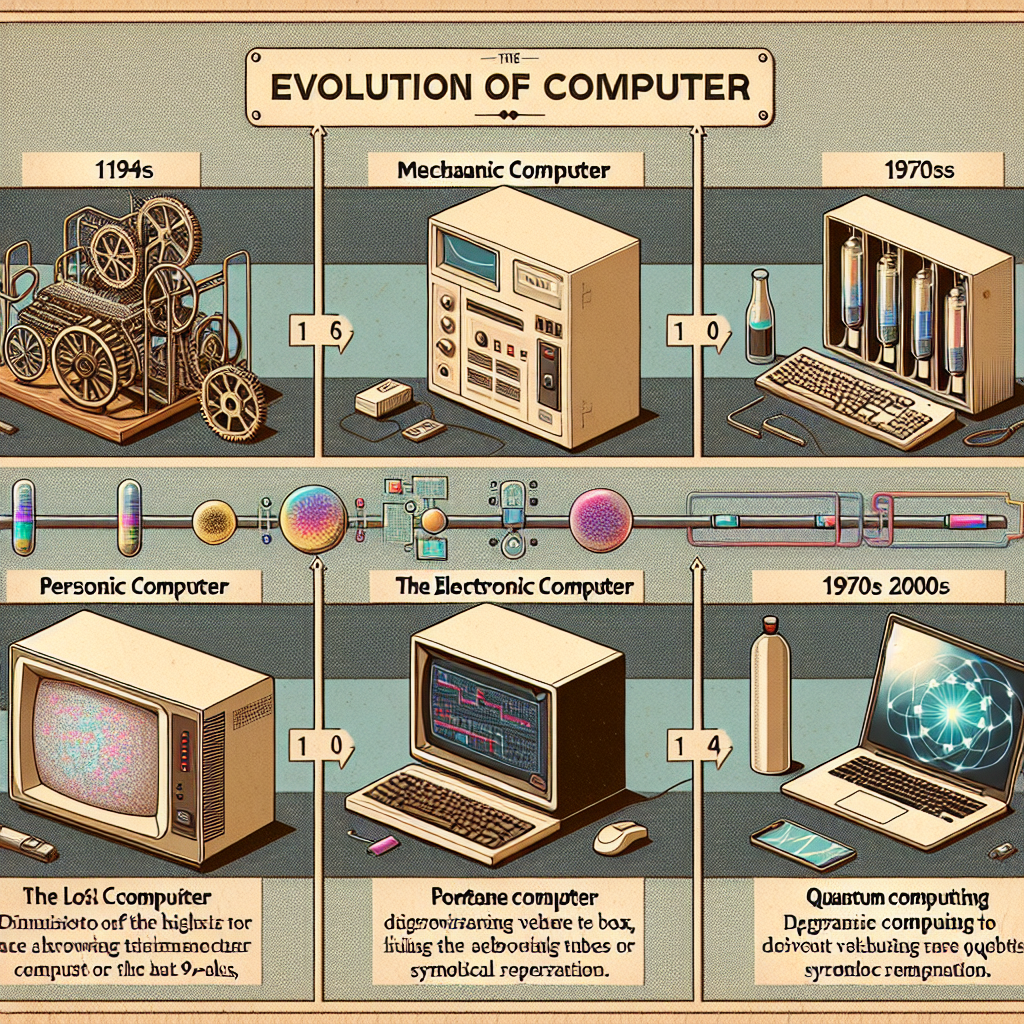The image is a detailed graphic artwork that appears to be a flyer or information sheet titled "The Evolution of the Computer," displayed in a white banner with black text at the top. The layout consists of six distinct illustrations, each depicting a different stage in the development of computers.

On the top left, the illustration is labeled "1194s" and features a tan-colored device with numerous round gear wheels, reminiscent of early mechanical computers. Adjacent to this image is another labeled "Mechanical Computer," showcasing a large, white box-like device with gear mechanisms and two small devices beside it.

Moving to the right, there is an illustration from the "1970s" depicting a vintage electronic computer. This computer is a white, square 3D design, featuring buttons on the front and a small blue screen on the top left, alongside a keyboard.

The lower row starts on the left with an illustration labeled "Persona, Personic Computer," which resembles an old TV screen and is partially obscured by unreadable text that mentions "The Lost Computer." 

Next to it, labeled "The Electronic Computer," is another boxed device coupled with a keyboard, again accompanied by some unreadable text beneath it. 

The far-right section covers "1970s to 2000s," portraying the progression towards modern computing devices like laptops and smartphones. It includes an image of a laptop, an iPhone, and what appears to be a water bottle, captioned "Quantum Computing." The entire piece uses a cold color palette, lending it a newspaper-like feel.